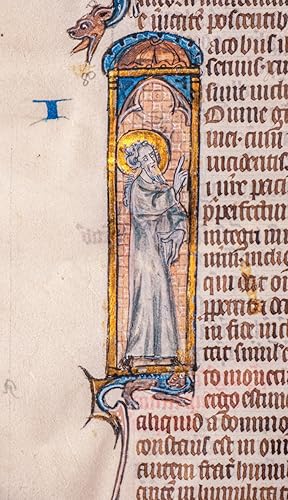The image, a detailed zoom-in on an illuminated manuscript, features an old drawing from what appears to be a book or scroll with a beige background. Dominating the center of the image is a tall, thin rectangular depiction of an old man, likely a saint, who is looking up at the text to the right. The man, clothed in a white robe with long wavy hair and a significant beard, is encircled by a yellow halo. He stands within a golden box highlighted by a brighter blue hue. His right hand is raised with a finger pointing upwards while his left hand holds something down. 

Surrounding him are patterned tiles in shades of dark and light pink, possibly simulating the appearance of a stained glass window. Above him is a semi-circular blue dome-like structure with gray below it, indicating the perimeter of a stained glass window. The top of the image features a dragon-like creature with a dark brown head and a dark blue neck, its mouth open and tongue sticking out towards a prominent blue eye in the margin to the left of the text.

The manuscript text, written in an unreadable Gothic font that is likely Latin, occupies most of the right side of the image. The margins also include a blue letter 'I'. At the bottom of the image, a dragon’s head, similar to the one at the top, adds to the mystical aura of the manuscript. This intricate and colorful composition, with its biblical semblance, illustrious saintly figure, and detailed patterned decorations, suggests the document is of significant cultural or religious importance.